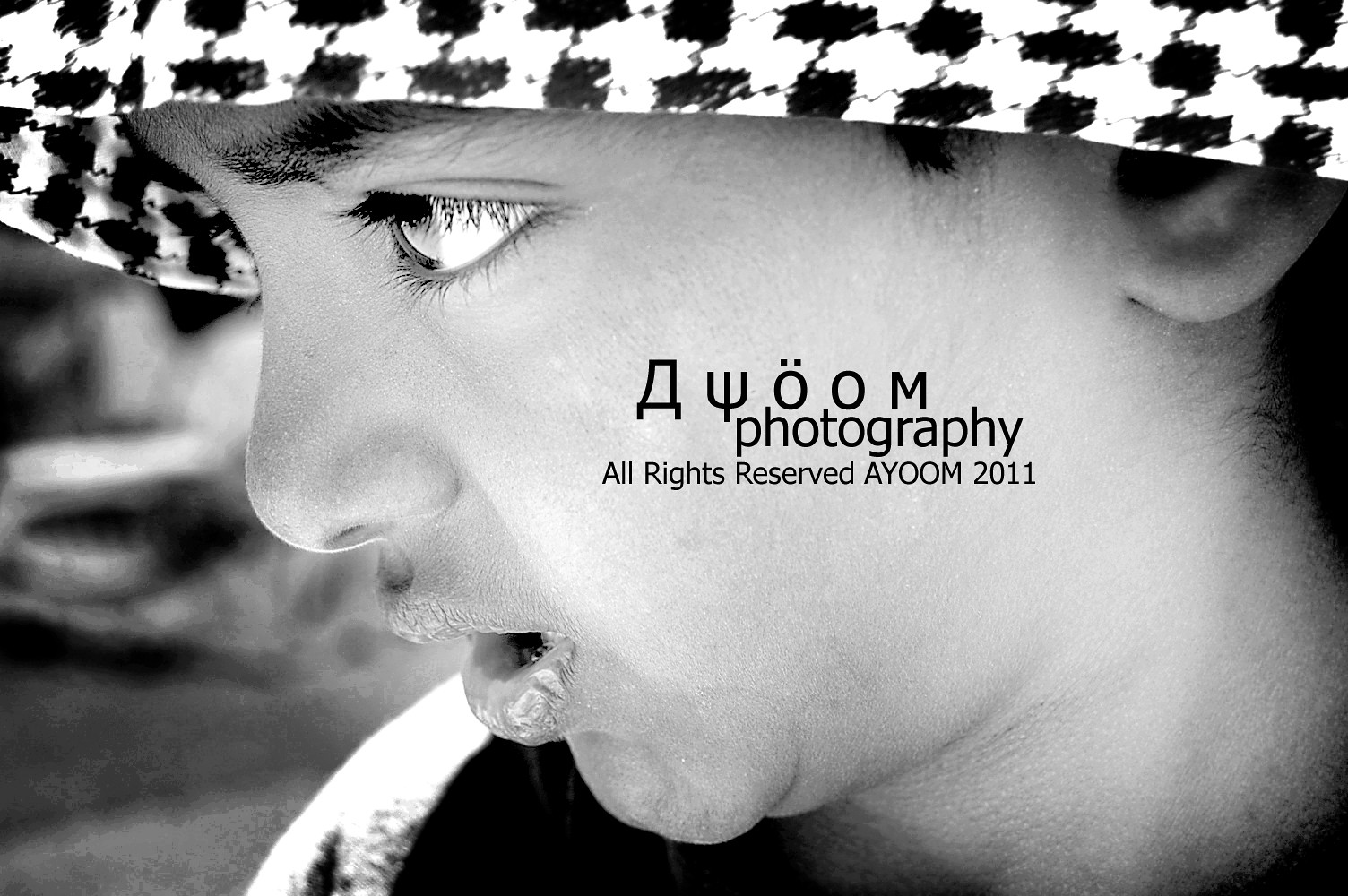This promotional black and white photograph from Aume Photography, copyrighted in 2013, features a close-up of a young boy, possibly between six to eight years old, looking towards the bottom left of the image. The boy's attire includes a distinctive black and white herringbone-pattern bucket hat, which obscures much of his head. He is also wearing a long-sleeve t-shirt, of which only the shoulder is visible. The boy's mouth is open, revealing lips that appear chapped and covered in a wet substance. His facial features include thick black eyebrows, long eyelashes, and a slightly sloped nose, with a portion of his lower earlobe peeking out from under the hat. The background of the image is very blurry, rendering it indistinguishable. Superimposed on the photograph is text in Greek, alongside the words "Photography All Rights Reserved," with the company’s name stylized as "Aume 2013" across the boy’s left cheek. The image is presented in a landscape orientation, adding depth and professionalism to the composition.